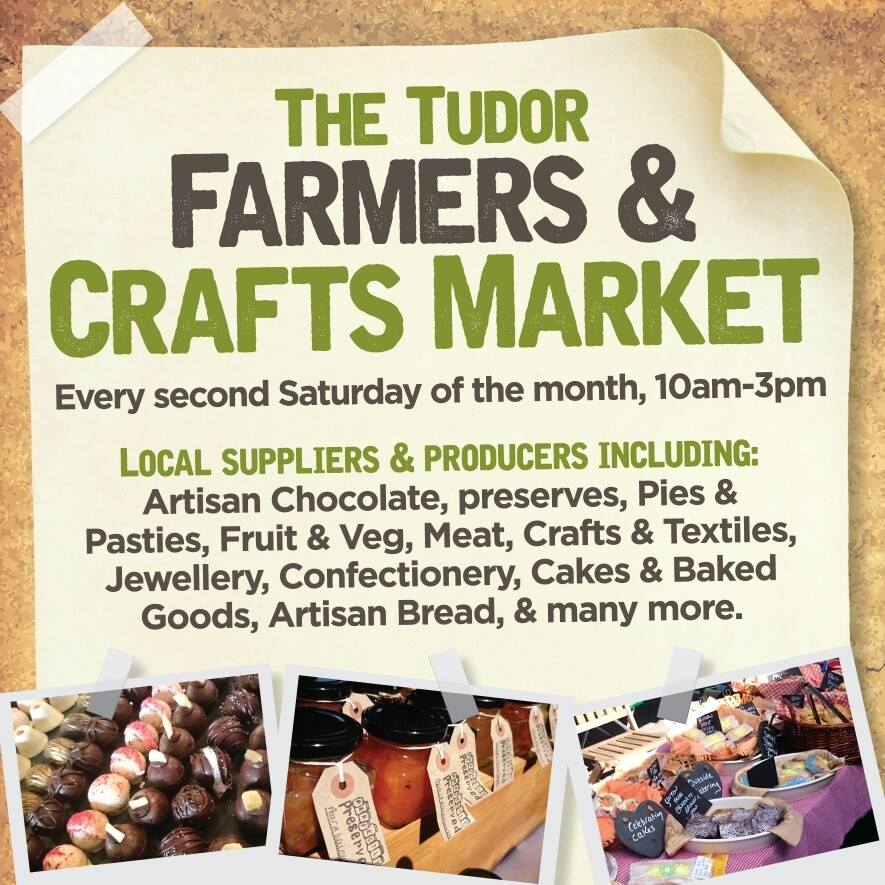This image depicts a flyer taped to a brown corkboard, advertising "The Tudor Farmers and Crafts Market." The flyer features a cream-colored background with green and black text. The event title uses green letters for "The Tudor" and "Crafts Market," and black letters for "Farmers." The subheading, also in black, reads "Every Second Saturday of the Month, 10am to 3pm." Below, in small green letters, it says "Local Suppliers and Producers Including," followed by a list in black letters: "Artisan Chocolate, Preserves, Pies and Pasties, Fruit and Veg, Meat, Crafts and Textiles, Jewelry, Confectionery, Cakes and Baked Goods, Artisan Bread, and many more." The bottom section of the flyer includes three images: the left picture showing brown and pink topped cupcakes, the center picture displaying jars of preserved fruit with black lids and tags, and the right picture presenting plates of various food items on a purple tablecloth. Notably, the flyer is attached with a piece of white tape, and the top right corner appears curled, giving it a slightly worn look.